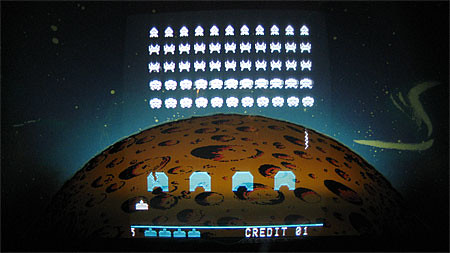This image is a color screenshot of a video game, likely "Space Invaders," presented within a rectangular frame oriented horizontally. The outer border of the frame is black. Inside the image, dominating the lower half, is a yellow, cratered planet that extends leftward and rightward from the center, fading into the black background. Scattered across the planet’s surface are numerous craters of varying sizes. 

Above this planet, the upper portion of the frame transitions into a dark blue sky, appearing to depict the universe. Within this sky area, ten alien creatures are arranged in five neat rows, clearly the eponymous Space Invaders, all uniformly white.

At the bottom of the image, there are four light blue, flat structures, which may serve as defensive mechanisms or bases. These structures have a distinct geometric shape, angling up the sides, across the top, and then down and under in a precise manner. The leftmost structure has a crack on its top left side. Just below these structures, in white text, is the label "Credit 01."